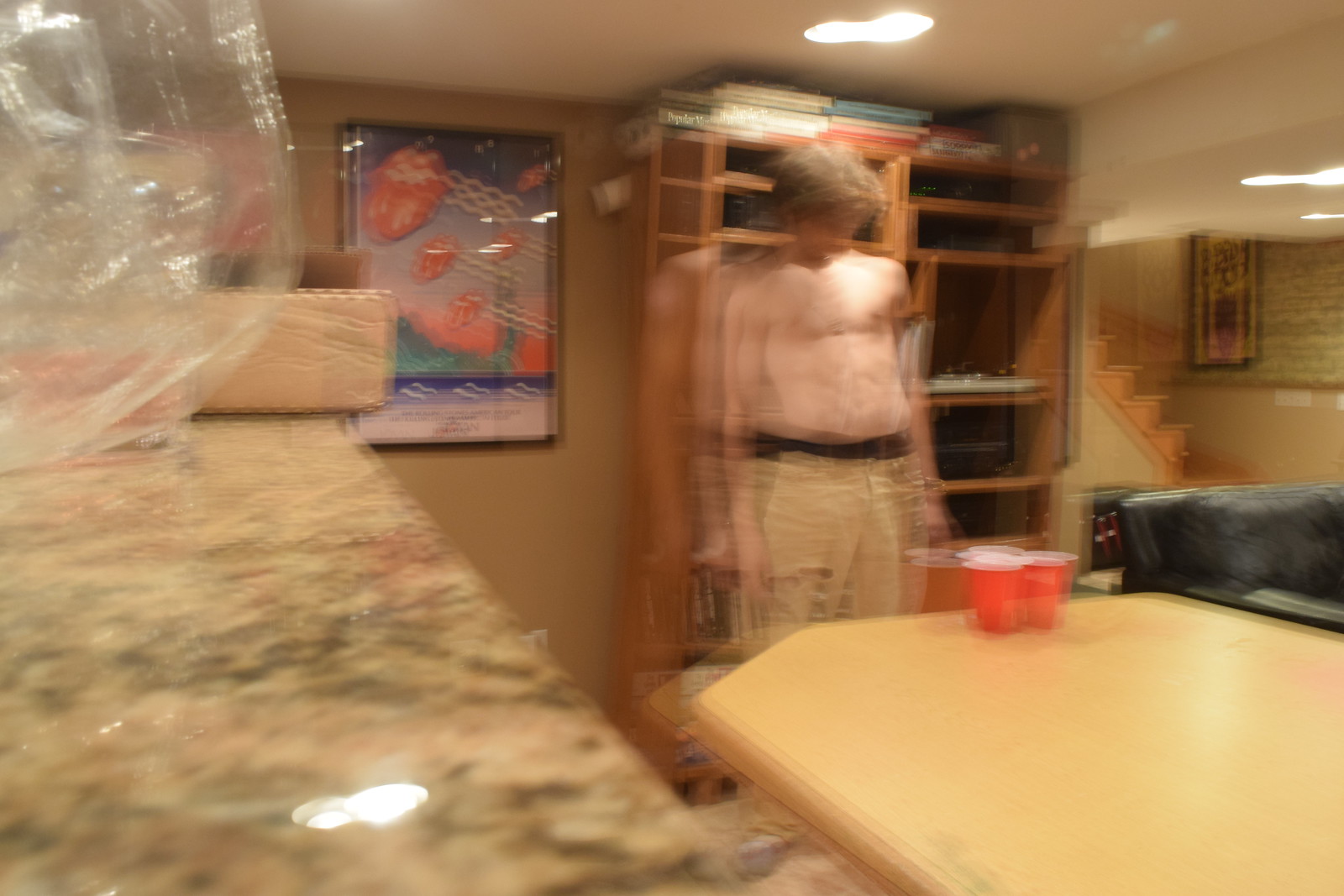A blurry photograph captures an individual standing shirtless in front of a beige table cluttered with red Solo cups. The person is wearing a belt and tattered, khaki-colored pants riddled with holes, giving off an unkempt appearance. Behind them, a set of stairs suggests the setting is a basement, possibly a den or recreational room. The background also features a shelf holding a turntable and a vividly framed Rolling Stones poster.